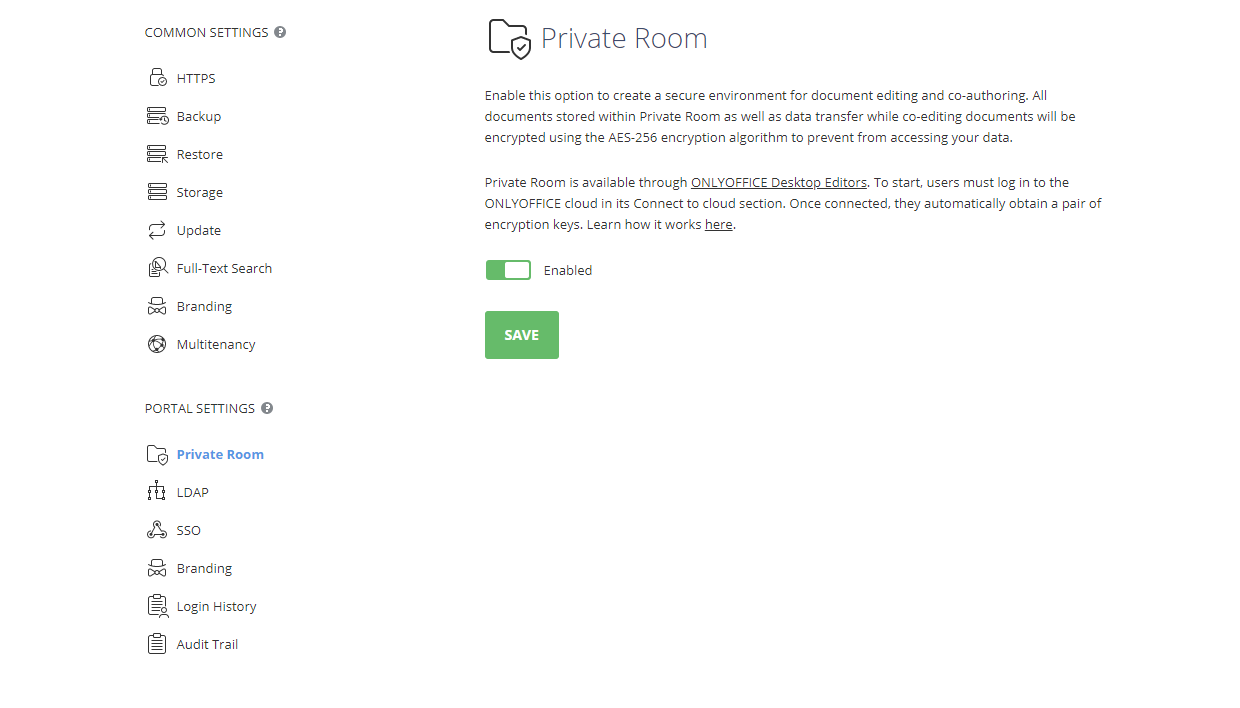In the image, a screenshot captured from a desktop screen showcases a user interface set against a white background. On the left side, a menu titled "Common Settings" is displayed in black text, listing various options: HTTPS, Backup, Restore, Storage, Updates, Full Text Search, Branding, and Multi Tenancy. Below that, a "Portal Settings" section is listed, including Private Room, LDAP, SSD, Branding, Login History, and Audit Trail, with all options in black text except for "Private Room," which is highlighted in blue.

Occupying the right side of the image is a detailed view of the "Private Room" settings page. The description explains, "Enable this option to create a secure environment for document editing and co-authoring. All documents stored within Private Room, as well as data transferred while co-editing documents, will be encrypted using the AES-256 encryption algorithm to prevent unauthorized access to your data." It also specifies that "Private Room is available through ONLYOFFICE Desktop Editors." Below the text, two buttons are available: one labeled "Enable" in white, and another labeled "Save" in green.